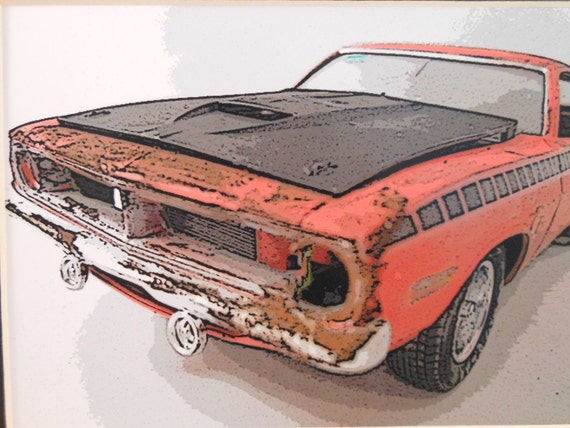The image depicts an old, classic red muscle car that has a highly detailed and stylized appearance due to a grainy, cell-shaded filter applied to it. The car, which is viewed at an angle focusing on the rusty front grill and the front left tire, has a significant amount of rust and dirt, especially on the front area. The black hood of the car contrasts sharply with its red body, which features black dots along the sides and what appear to be silver elements, possibly missing headlights. The windshield is dirty, obstructing the view through it, and has a blue sticker on the upper right corner. The entire car is immersed in a washed-out, pixelated filter, set against a stark white background, suggesting a stylized photographic technique reminiscent of Photoshop's stroke action effect. The car, possibly a hot rod or a Mustang, has a distinctive stripe of squares along its side, further accentuating its classic, rugged appearance.